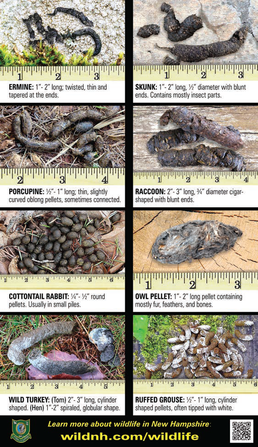This infographic showcases eight different types of wildlife droppings, each labeled with the corresponding animal's name, measured by rulers beneath the images. The left column features droppings from an ermine, porcupine, cottontail rabbit, and wild turkey. The right column displays feces from a skunk, raccoon, owl pellet, and ruffed grouse. Each image includes a detailed description of the feces, highlighting characteristics such as length and color. At the top of the chart, a black bar names the animal that produced the dropping, while at the bottom, another black bar with yellow text invites viewers to "learn about wildlife in New Hampshire" at wildnh.com/wildlife. Additionally, a QR code is provided for quick access to more information.